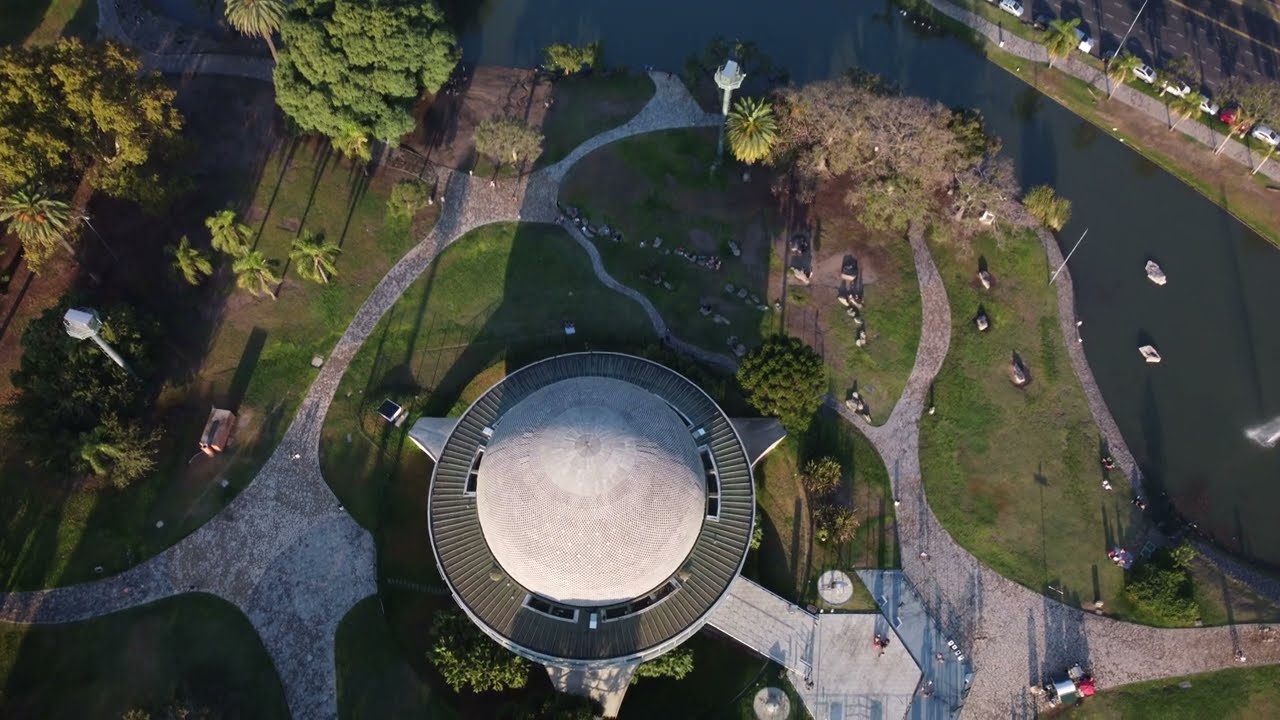This aerial, bird's eye view photograph reveals a sunny landscape featuring a circular, dome-style building. The building's roof, a concrete dome, is accentuated by wooden slats and skylights that encircle its structure. Leading to and from the edifice are multiple concrete pathways, meandering through a well-maintained green lawn adorned with trees and bushes. Scattered across the property are a few people, leisurely milling about. Adjacent to the building lies a picturesque body of water, possibly a canal, where a few boats can be seen. Across from this waterway, several cars are parked neatly along a street, casting shadows in the sunlight that highlights the depth and contours of the scene.